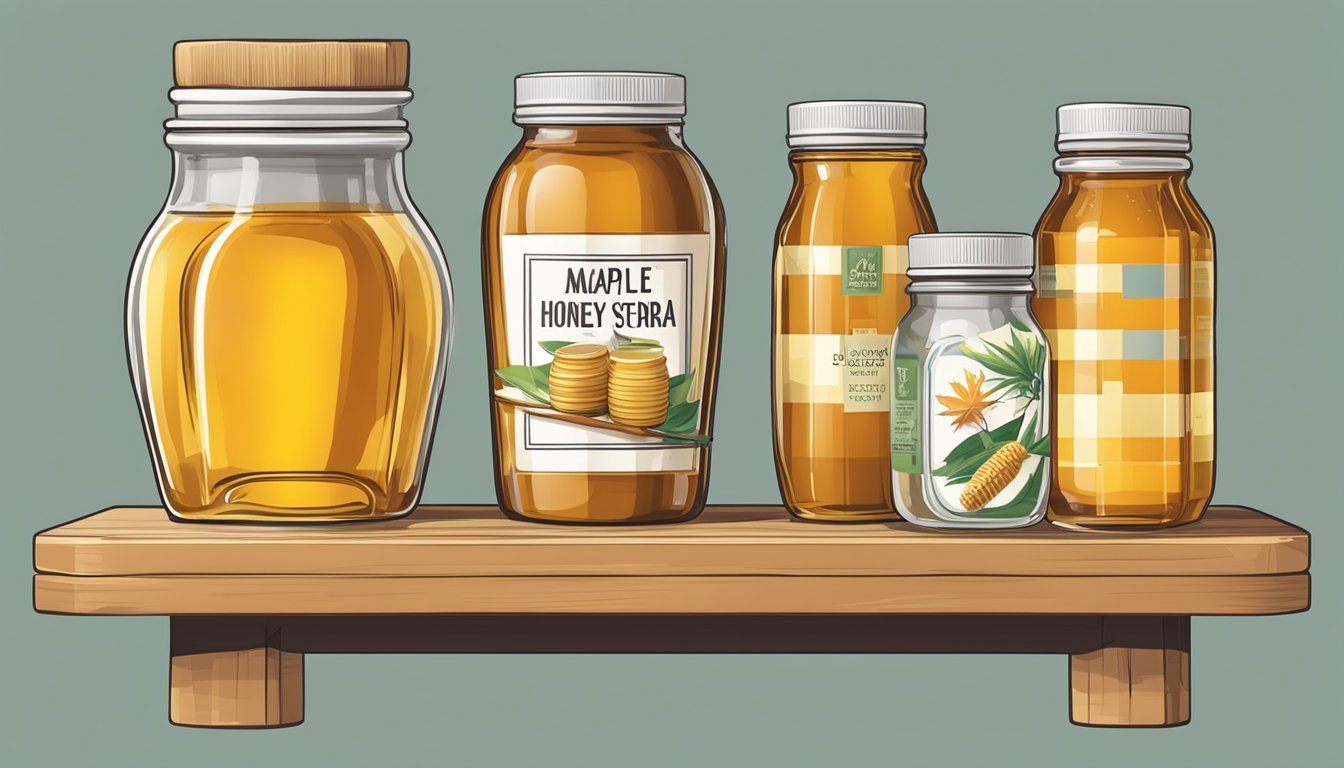The digitally created image features a horizontally aligned, rectangular frame with a solid, lighter green background. Mounted against this background is a wooden shelf with two short legs, appearing to hold the shelf in place. The shelf houses five glass jars, each varying in size and content.

On the far left is the widest jar, a clear glass container with a wooden lid, appearing to contain a golden liquid, likely syrup or honey. Adjacent to it is a slightly narrower but equally tall jar with a silver lid. This jar features a label reading "maple honey syrup" along with an illustration of a stack of pancakes. Following that is another similarly tall but narrower jar with a silver lid, filled with what seems to be a golden liquid.

To the right of these, there is a smaller jar with an image of leaves on its front and appears to be empty or filled with a clear liquid. Finally, the jar on the far right is taller with a silver lid and has a distinctive checkered pattern in gray and gold.

The arrangement and varying designs of the jars, combined with the simple wooden shelf and the solid green background, create a charming and cohesive visual composition.